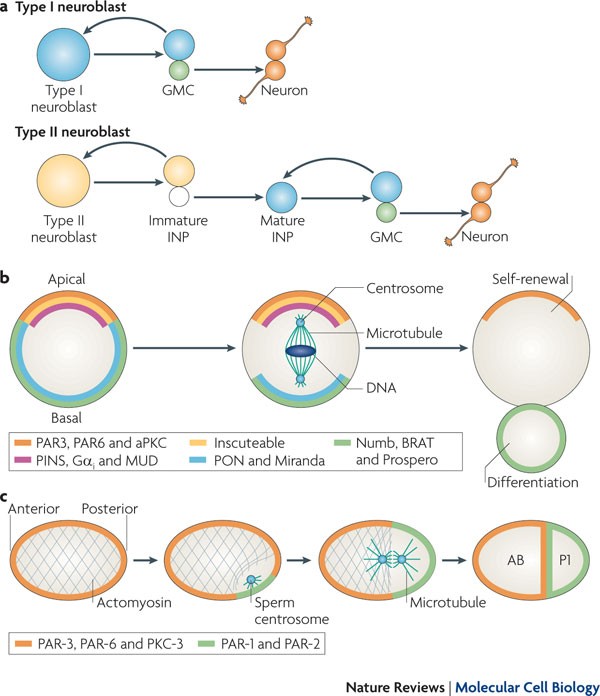The image, sourced from "Nature Reviews Molecular Cell Biology," is a detailed and vibrant educational chart divided into three sections labeled A, B, and C from top to bottom. Each section outlines different aspects of cellular biology, with a focus on neuroblasts.

**Section A:** This section depicts the development of neuroblasts, displaying the differentiation pathways of Type 1 and Type 2 neuroblasts. It shows Type 1 neuroblast (labeled in blue) leading to a GMC (ganglion mother cell) and eventually to a neuron. Similarly, Type 2 neuroblasts (represented in orange) proceed through stages of immature INP (intermediate neural progenitors) and mature INP, sequentially transforming into a GMC and finally a neuron. Detailed labels include "GMC" and "Neuron," with colored dots (orange, blue, green) marking various stages and connections.

**Section B:** This section highlights cellular components and processes associated with cell self-renewal and differentiation, presenting terms like "Apical," "Basal," "Centrosome," "Microtubule," and "DNA." It emphasizes the concepts of polarity and the molecular machinery involved in these processes. Various proteins and complexes are color-coded: orange for Par3, Par6, and aPKC; purple for Pins, Gα, and Mud; yellow for Insc; blue for PON and Miranda; and green for NUM, Brat, and Prospero.

**Section C:** This section focuses on cell polarity and spatial organization, elucidating "Anterior-Posterior" orientation, "Actomyosin," and the roles of "Sperm Centrosome" and "Microtubule." It labels structures like "AB and PI" inside ovals and reiterates key proteins such as Par3, Par6, PKC3, as well as Par1 and Par2. 

Overall, the chart is brightly colored, well-lit, and clear, providing a comprehensive view of neuroblast differentiation and cellular polarity mechanisms.